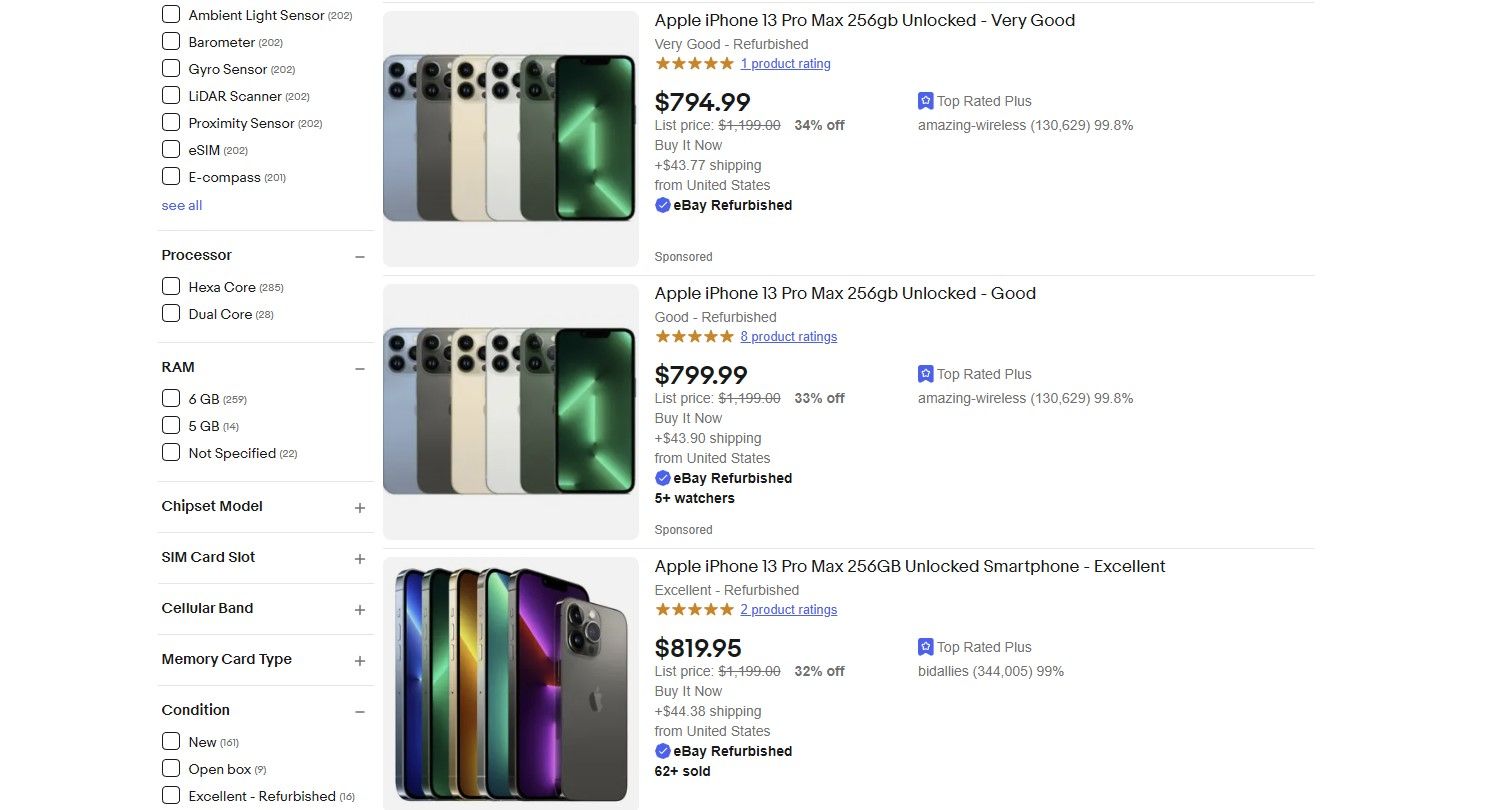A detailed screenshot of an Apple refurbished iPhones listing on eBay. The page is divided into three distinct sections, each separated by a thin gray line, showcasing various refurbished iPhone models in differing conditions. 

On the left side, an interactive menu allows users to filter options by color, condition, memory capacity, RAM, and processor type. The center section prominently features images of the iPhones closely aligned to display the available color variations. To the far right, detailed descriptions provide essential information about each iPhone, including its condition, price, specific model, and series. 

At the bottom of each listing description is a blue checkmark symbol indicating that these devices are eBay Certified Refurbished.